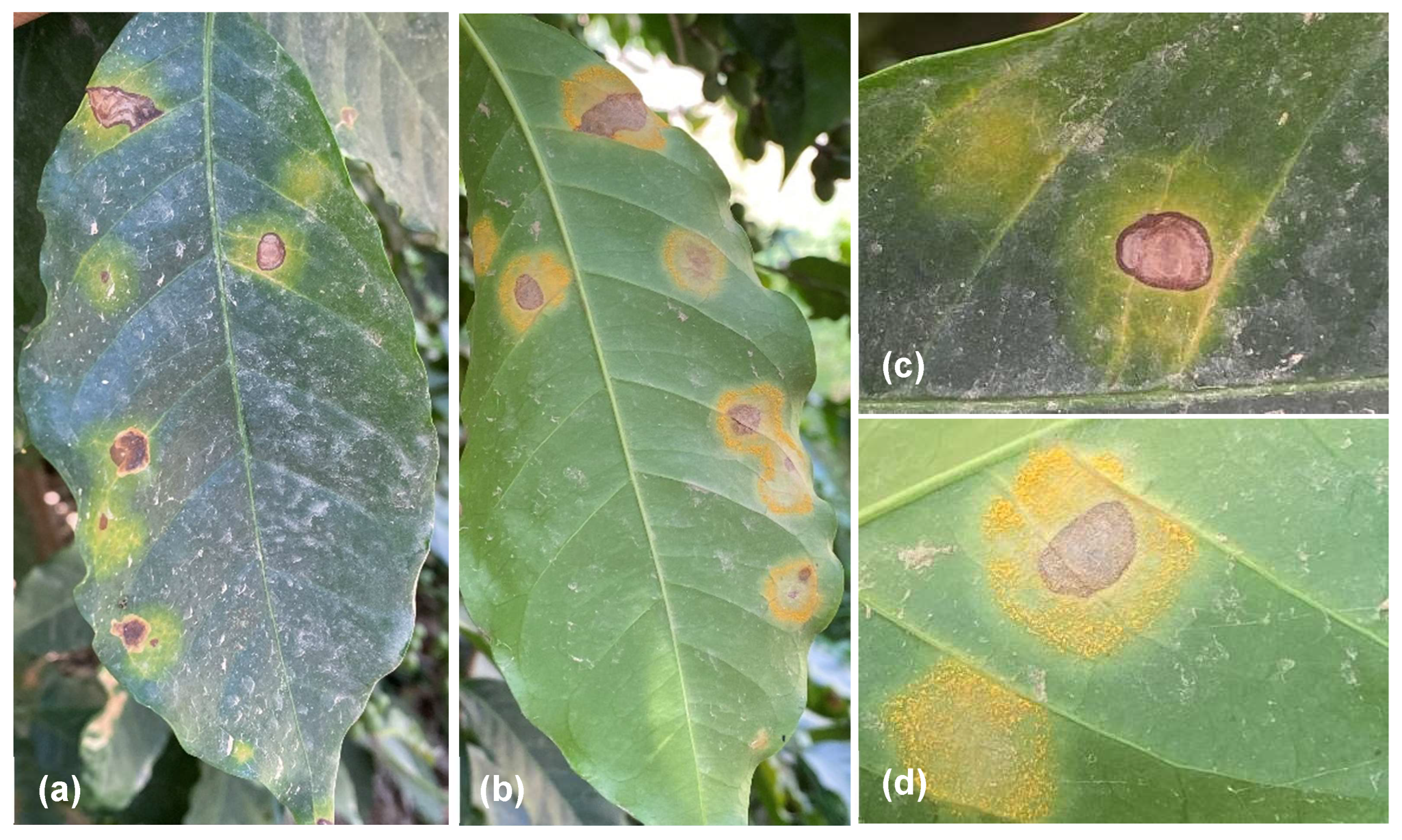The image is a four-part collage, labeled A, B, C, and D, showcasing leaves with various stages of brown and yellow spots, indicative of damage or disease. The collage is divided into two vertical rectangles (A and B) on the left and two stacked horizontal squares (C and D) on the right. Image A features a non-close-up view of a green leaf with several brown spots, suggesting early signs of decay. Image B displays a similar leaf, slightly healthier but still with visible brown and yellow spots. Images C and D are close-ups of the leaves shown in A and B, respectively, providing detailed views of the brown spots. The leaves are depicted with dull green hues and numerous surface-level spots, appearing unhealthy but not entirely dead.